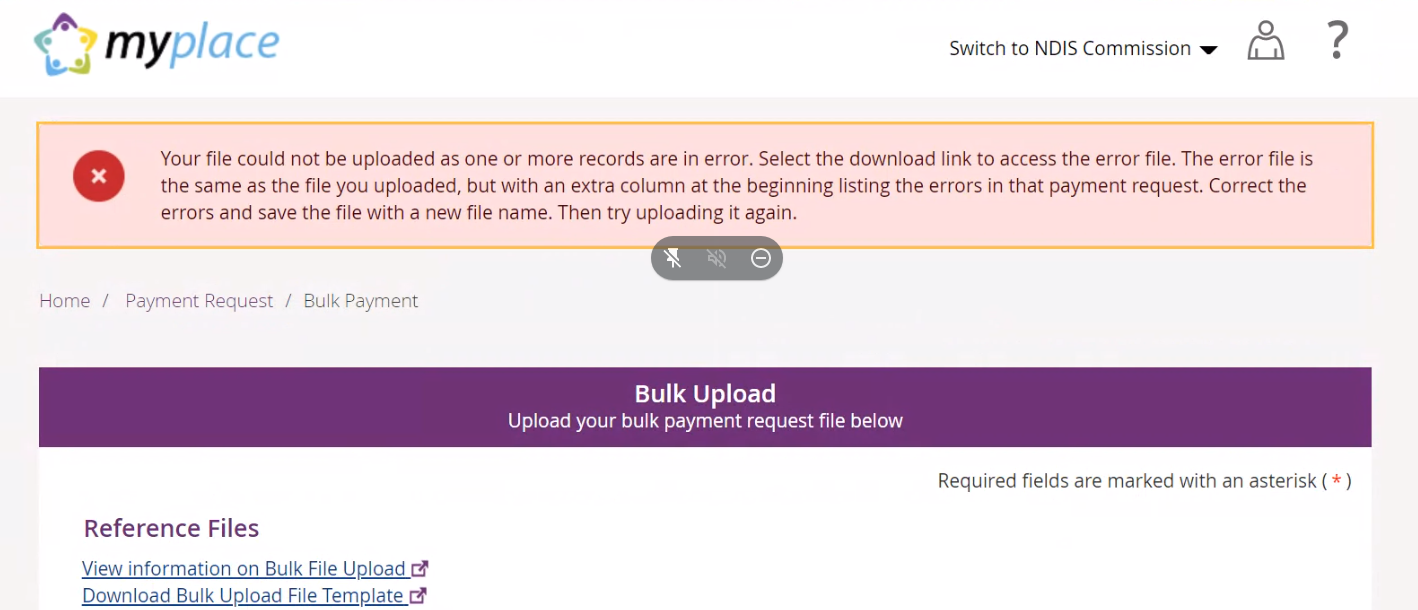This image, a screenshot of a website interface, features several key elements. At the top left, there is a multicolored five-pointed star icon followed by the words "my place"—with "my" in black and "place" in blue. To the right, black text reads "switch to NDIS commission," accompanied by a downward arrow, a figurine of a person, and a question mark icon.

The website has a gray background. Below the top section, there's a prominent pink box outlined in orange. On the left side of this box is a red circle with a white "X" inside. The text within the pink box, in black letters, states: "Your file cannot be uploaded as one or more records are in error. Select the download link to access the error file. The error file is the same as the file you uploaded but with an extra column in the beginning listing the errors in that payment request. Select the errors and save the file with a new file name, then try uploading it again." 

Centered below this pink box is a small black tab featuring three icons: a pin with a strike-through, a speaker with a strike-through, and a white circle with a line through it.

Underneath the pink box on the left, black text reads: "home/payment request/bulk payment." Below that, there is a purple bar with white text that says "bulk upload," which is highlighted. The instructions "Upload your bulk payment request file below" are also included. The purple bar extends down into a white box. On the left side of this white box, purple text reads "reference files." Beneath this are two blue, underlined links: "view information on bulk file upload" and "download bulk upload file template."

On the top right, just below the purple section, there is a note that states: "required fields are marked with an asterisk," followed by a red asterisk in parentheses.